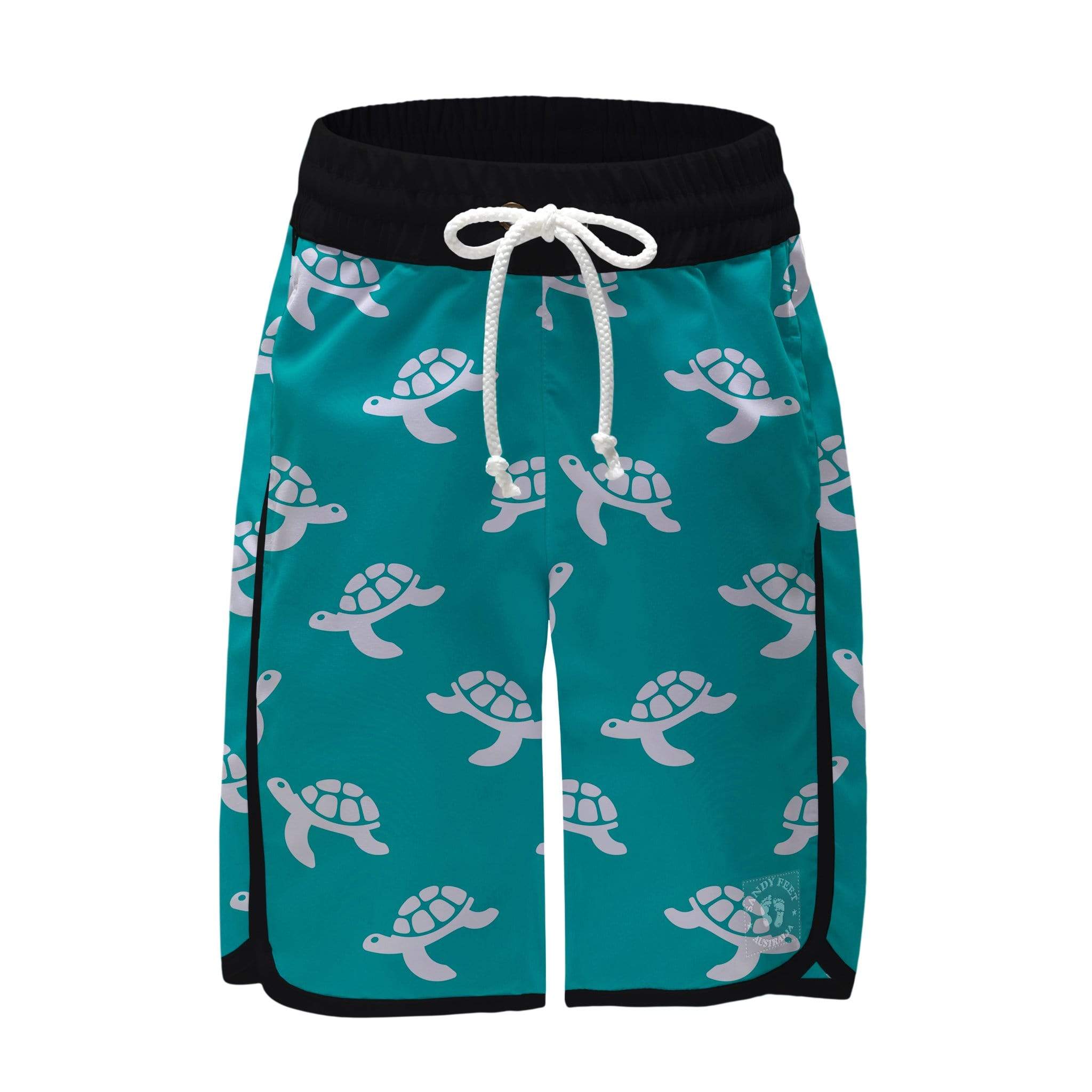This close-up image showcases a pair of swim trunks against a completely white background. The swim trunks feature a vibrant turquoise base color adorned with white sea turtle prints, each turtle facing different directions in a repetitive descending pattern. The trunks are designed with a black waistband and a white drawstring at the center, tied in a small loop, with the ends hanging down. The legs of the trunks extend down to the knees, bordered by a sleek black trim that runs along the bottom and up the sides toward the pockets. Each side of the trunks has a pocket. On the bottom right leg, there is a logo that reads "Sandy Feet Australia" accompanied by two small footprints.